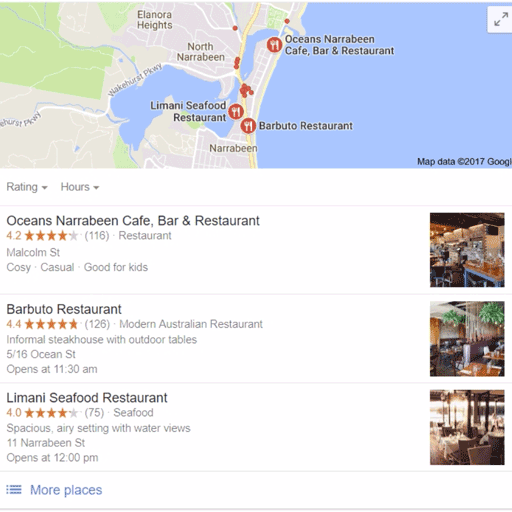**Screenshot of a Restaurant Search in North Narrabeen: Detailed Description**

The screenshot captures a person searching for dining options in North Narrabeen and neighboring areas, including Eleanora Heights. The map, sourced from Google (copyright 2017), displays notable locations such as Oceans, Narrabeen Cafe, Bar, and Restaurant. 

Highlighted restaurant selections include:

1. **Malcolm Street Cozy Casual**: This kid-friendly eatery boasts a rating of 4.2 stars from 116 reviews. It's characterized as a casual restaurant located at Malcolm Street, ideal for family outings.

2. **Barbuto Restaurant**: With a commendable rating of 4.4 stars from 126 reviews, this Modern Australian Restaurant offers an informal steakhouse experience with outdoor seating. It's situated at 516 Ocean Street and opens at 11:30 a.m.

3. **Lamali Seafood Restaurant**: This spacious, airy establishment enjoys a scenic water view and specializes in seafood. It holds a 4-star rating based on 75 reviews and opens at noon. It's located at 11 Narrabeen Street.

The screenshot includes a blue context menu at the bottom for exploring more dining places. The image also details a sleek bar and a very fancy restaurant, noted for its visually striking setting with textured red, white, and gray chairs as well as hanging plants, evoking an upscale yet inviting ambiance.